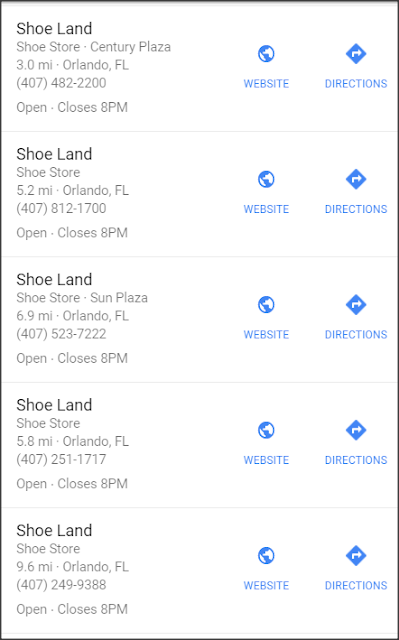A detailed caption for the image could be: 

"The image displays the search results for 'Shoe Land' locations in Orlando, Florida on a cell phone. The search itself was conducted off-screen, and five 'Shoe Land' stores are listed on the visible screen, each entry containing comprehensive details. For each store, the address is clearly indicated, as well as the specific shopping mall or plaza it resides in, the distance from the searcher's current location, a contact phone number, and the store's opening and closing hours. On the right side of the screen, there are two vertical columns with blue icons and text. The first column features clickable 'Website' buttons for each store, while the second column provides 'Directions' buttons for easy navigation to the selected location."